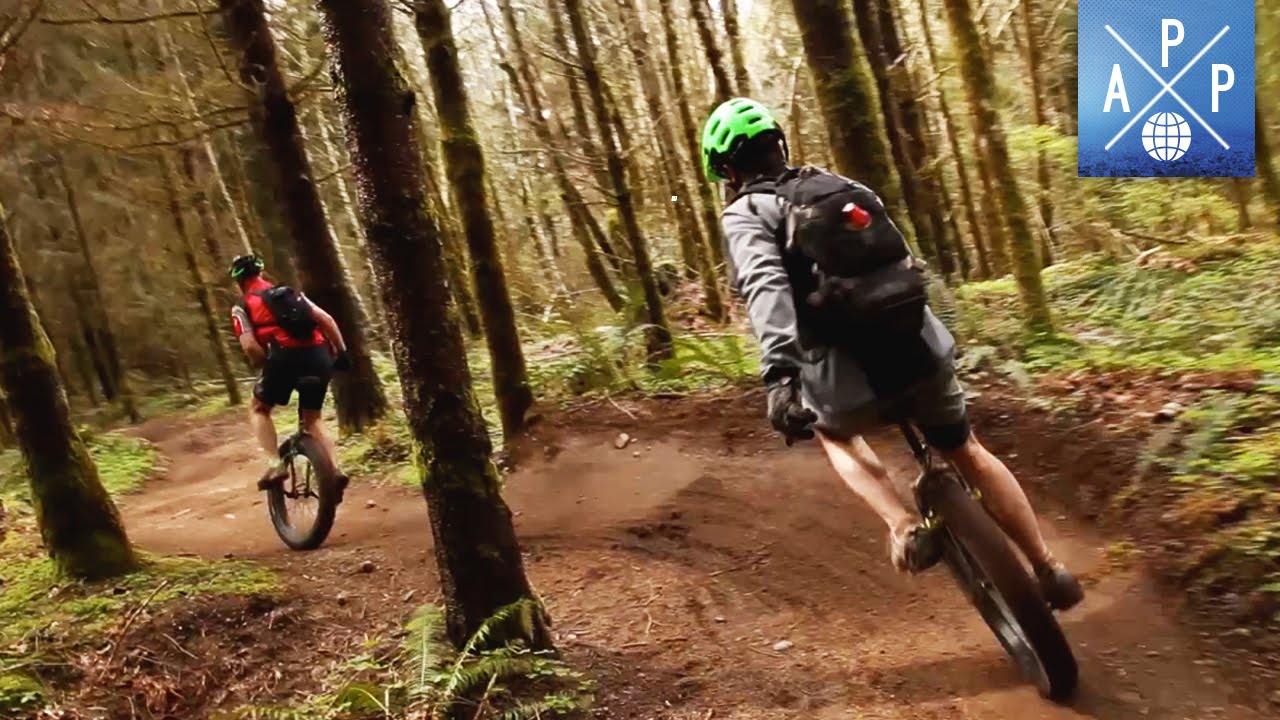This photograph captures an action-packed scene of two men riding unicycles along a winding dirt trail through a forest. The trail, well-worn and devoid of rocks, stretches out in a meandering path, flanked by small to medium-sized trees and a variety of greenery, including ferns. The rider closest to the camera is wearing a green protective helmet, black backpack, black shorts, and visible gloves, exuding a sense of focus and intensity. Ahead of him, the second rider sports a black helmet, red shirt, and black shorts, and appears to glance to the left, maintaining his balance on the narrow, marked-out trail. Both riders are equipped with helmets, backpacks, and are bare-legged from the knees down, indicating that they are probably tackling this forest trail on a cooler yet clear daytime, devoid of any text overlay on the image. The background is rich with blurred foliage, enhancing the sense of movement and speed. The overall composition suggests a thrilling and adventurous moment, as the two men navigate the picturesque yet challenging path.